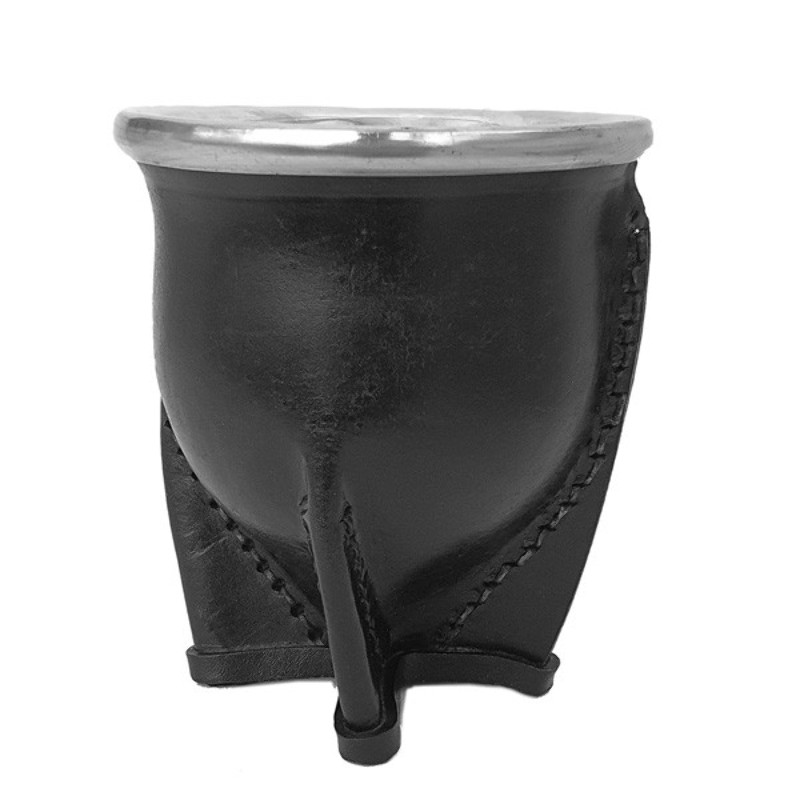The image captures a uniquely shaped object that resembles a cup or bowl, featuring an interesting blend of materials and design elements. The lower part of the object is encased in black leather, meticulously stitched together to form a plus-sign-shaped base that provides stability. This woven leather casing tightly envelops the bottom section, adding a decorative yet functional aspect. The top portion of the item is circular, made of a shiny, metallic silver material. The rim is visible, but the interior cannot be seen, making it unclear whether the top is solid or concave, as expected in a traditional cup. The white background enhances the focus on the intricate details of the black leather stitching and the contrast between the leather and the silver metal. While its precise function remains ambiguous, the object combines aesthetics with utility, suggesting it as a potential decorative daily-use item, albeit one that may not withstand regular washing due to the leather components.